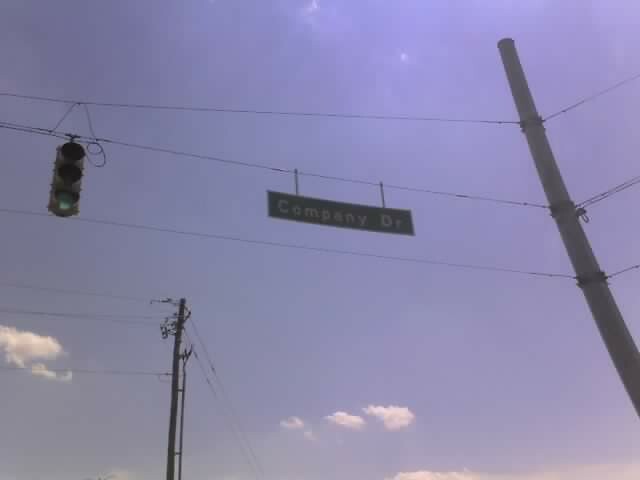The photograph captures a rather puzzling scene on a seemingly sunny day, despite a noticeable haze that suggests air pollution. The sky is predominantly blue, peppered with a few white clouds towards the bottom and a tiny bit at the top of the image.

On the lower left-hand side, there is a tower that doesn’t quite resemble a typical telephone pole, but it might be, considering its distant placement. A network of wires extends from this tower; some veer off to the left, while a few stretch diagonally downward to the right.

On the right-hand side of the image, another pole stands tall. Initially it appears to be a wooden telephone pole, but upon closer inspection, it seems to be a circular metal pole. This pole supports three lines of wires branching out both to the right and left. 

The lowest wire on the left side curiously lacks any visible attachments. The middle wire, however, has a street sign hanging from it that reads “Company Drive,” though its color remains indiscernible. Further to the left, there is a streetlight with a faintly visible green light, adding to the mysterious haziness of the scene. The upper wire doesn’t have any direct attachments, but it does bear part of a traffic light whose wire loops over it. 

Altogether, the image weaves a curious intersection of urban elements set against an unusually hazy sky that masks the sunlit clarity one would expect.